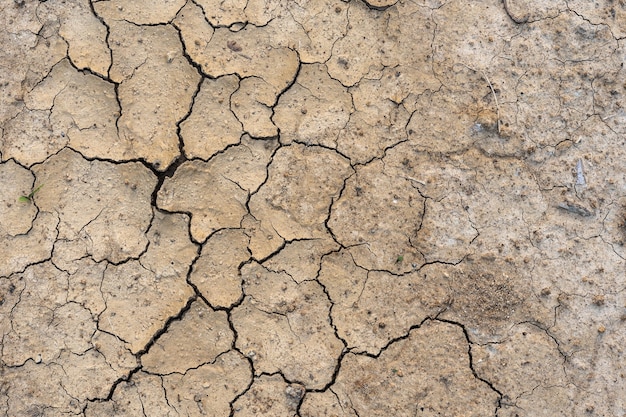The image depicts an arid landscape with severely cracked soil, indicative of extreme drought conditions. The earth's surface is fractured extensively, with large, deep fissures running throughout the terrain. On the right-hand side, the ground is so desiccated that it appears bleached, exhibiting a stark white hue. The left side is even more parched, emphasizing the severe lack of moisture. There is no vegetation visible, save for a single dead weed, highlighting the absence of any substantial plant life. The scene lacks any water bodies or other environmental features, focusing solely on illustrating the extent of the soil's dehydration. This close-up perspective underscores the harsh reality of dry land.